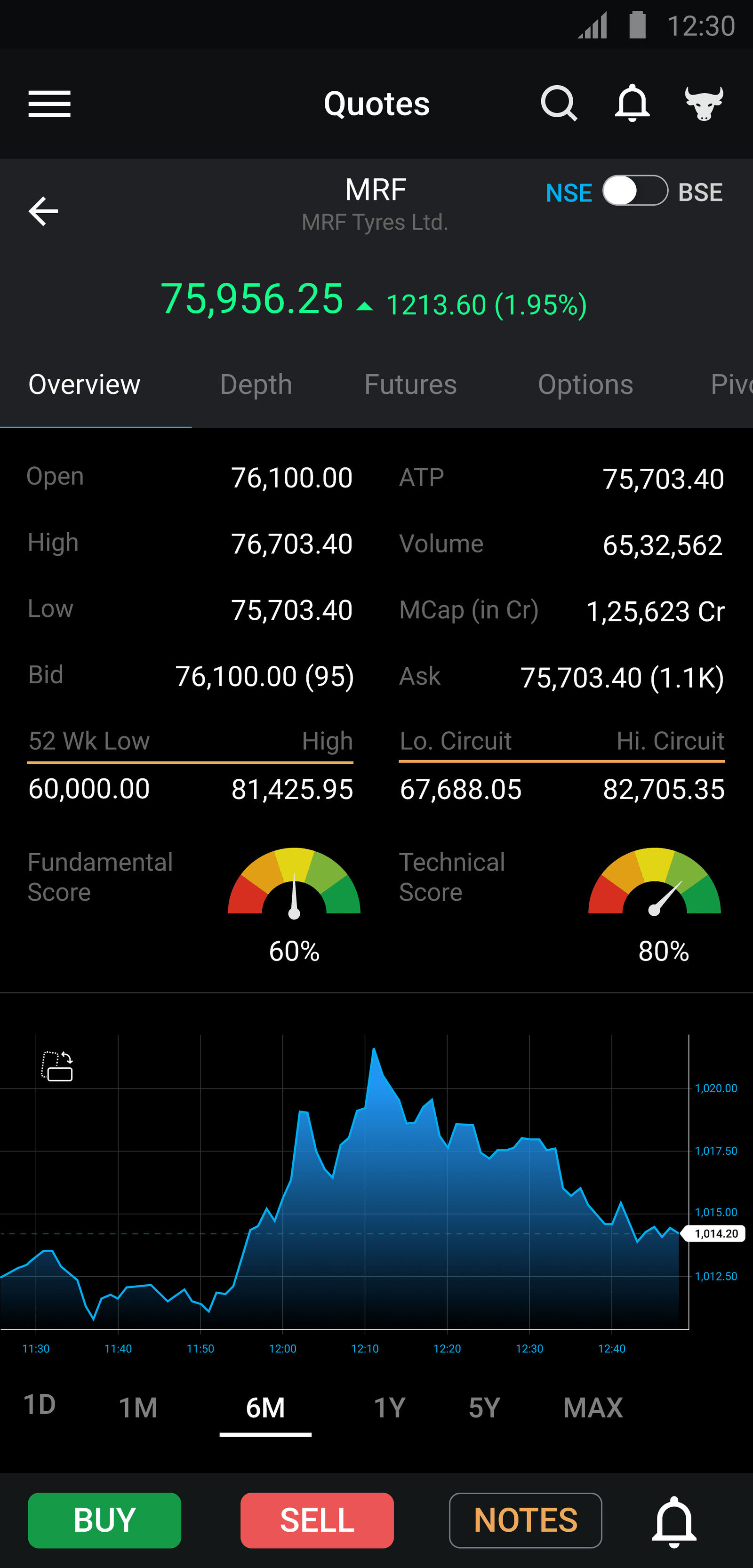The image is a detailed screenshot of a trading app interface, featuring various trading and information elements. On the lower left, there are 'Buy' and 'Sell' buttons, with the 'Buy' button in green and the 'Sell' button in an off-red color, both with white, all-caps lettering. Adjacent to these buttons is a ‘Notes’ button, displayed in an off-orange color with a black background. To its right, there is a white bell icon.

At the bottom of the screen, a graph is displayed with timeframes such as 1D, 1M, 6M, 1Y, 5Y, and MAX, representing day, month, six months, year, five years, and a maximum timeline for the data shown. Above this graph, the screen presents various financial indicators including a fundamental score of 60% and a technical score of 80%. It also details the stock's open price, high and low prices, bid price, 52-week low and high, and both low and high circuit limits.

The app's menu featuring options like 'Overview', 'Depth', 'Futures', and 'Options' is located above these statistics. Further up the screen, the current value of a particular stock is shown as 75,956.25, with an upward-pointing arrow indicating an increase of 1213.60 (1.95%). The stock is labeled as MRF with additional labeling showing "MRF Tires Ltd" and 'Poyard'. 

In the upper-right corner, there are radio buttons labeled NSE and BSE, which likely stand for National Stock Exchange and Bombay Stock Exchange, respectively. Additionally, the typical status icons for time, battery life, and Wi-Fi signal are displayed, suggesting this app is being viewed on an Android device.